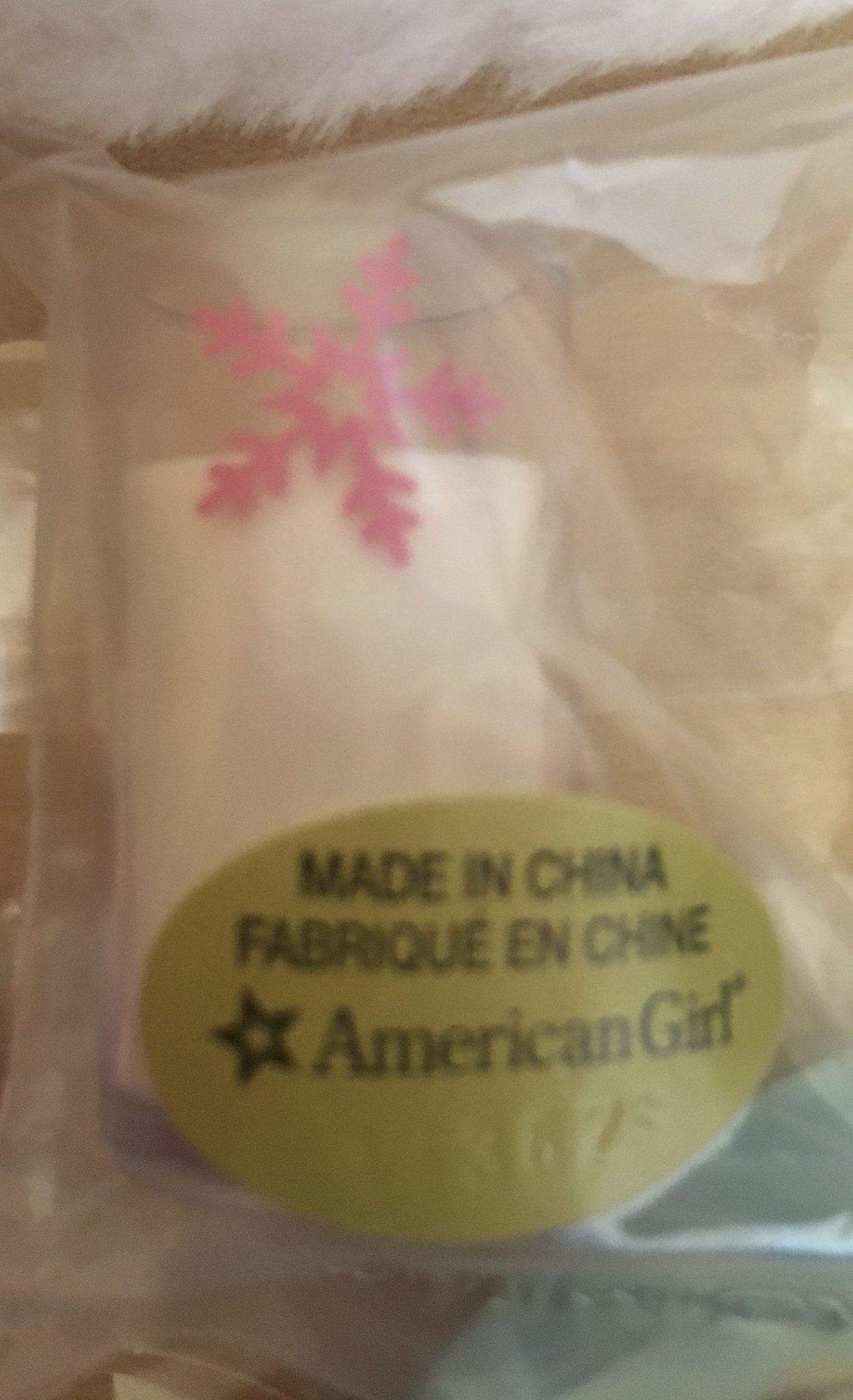The photograph captures a close-up of a discolored yellowish-brown clear plastic bag, centrally showcasing an American Girl product. The bag features a distinctive yellow oval logo in the bottom left, marked "American Girl." Above this, the label in black capital letters states "Made in China," followed by "Fabrique en Chine." The upper left corner of the bag is adorned with a pink star-centered snowflake. Inside the transparent plastic, a white rectangular object is visible, though its exact nature—possibly fabric or a roll of tape—remains unclear. The plastic bag's bottom is heat-sealed. The scene includes various background elements: a green, oval-like shape resembling a dish or paper plate in the lower half, and a wood-colored desk underneath. At the image's top edge, there is a fuzzy, fluffy white object, potentially a towel or blanket. The slightly out-of-focus and dimly lit image adds a layer of ambiguity to the bag's contents and surroundings.